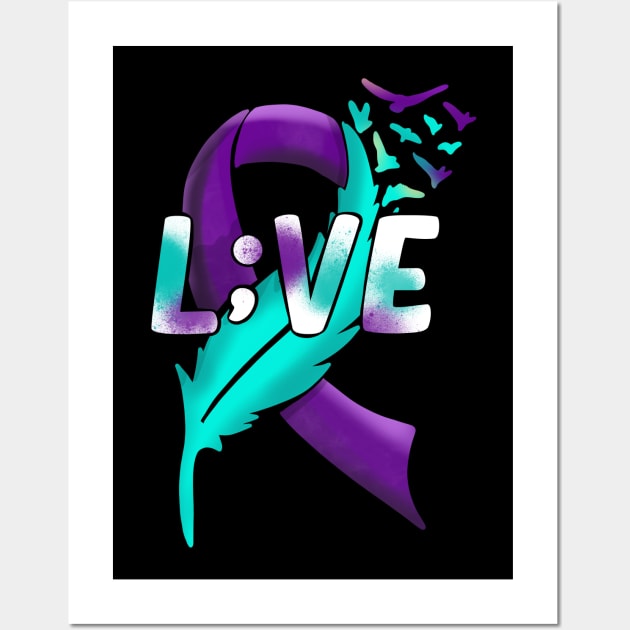The image depicts a highly stylized digital artwork featuring a multi-layered background and intricate details. The primary background is a solid grey, overlaid with a raised white rectangle that casts subtle shadows along its right and bottom edges. Within this white rectangle is a central black rectangle, creating a white border around it.

At the core of the design is a black sign bearing the text "L;VE," where the "L" and "E" are separated by a semicolon. These letters are prominently white and adorned with a spray-painted, tie-dye effect in shades of purple and teal.

Overlaying this text is a decorative element comprising a purple ribbon transitioning into a teal feather. This feather is illustrated with a unique, delicate pattern that includes alternating purple and teal birds. These birds appear to be taking flight from the top right corner of the feather, with some birds showcasing a blend of both colors, split half and half.

The image combines elements of typography and abstract art to create a visually engaging and symbolically rich composition, balancing vibrant colors with structured design elements.